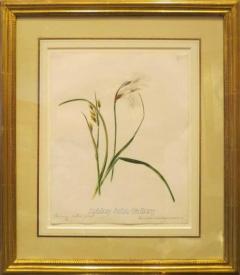This image is of a framed print, depicting an intricately detailed drawing of various grass stalks and seed pods, set against a light-colored background. The rectangular wooden frame, in a portrait orientation, is light brown with a gold matting inside. The picture itself is bordered by a tan margin which is adorned with a thin black line separating it from the central illustration. 

The drawing showcases multiple wispy stalks of grass or wheat. On the left, a green stalk curves upward and forms a backward 'C'. To its right, a tall blade of grass stands, adorned with two or three seed pods near the top. Adjacent to this stalk, another piece of grass arches to the left, resembling a Y-shape, with small seeds on the right side of the Y. Another stalk, characterized by a gentle downward swoop toward the bottom right-hand corner, adds movement to the composition.

Beneath the drawing, there is barely visible, faint script, possibly denoting a date like "April 1817," though the text is unclear. Overall, the framed piece combines natural elegance with historical charm through its delicate and detailed botanical representation.